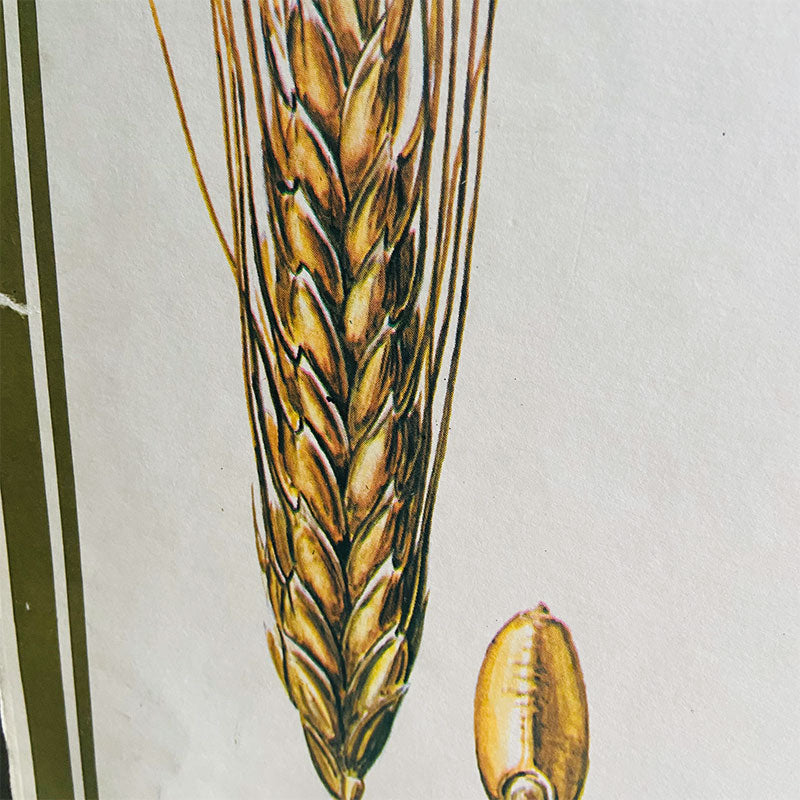This detailed illustration features a close-up of a golden bronze wheat plant arching gracefully from the bottom center of the image to the very top. Each kernel and the intricate threads of the wheat plant are meticulously detailed, showcasing the interlocking, criss-crossed pattern of the plant fibers. To the right of the wheat plant, there's a singular grain or seed, slightly out of focus, yet still noticeably matching the harvest yellow hue of the wheat. The background is a white solid gradient, suggesting that this detailed drawing, likely created with colored pencils, might be a page out of a school textbook. The image has a slight sage green border to the left, further framing the botanical illustration.